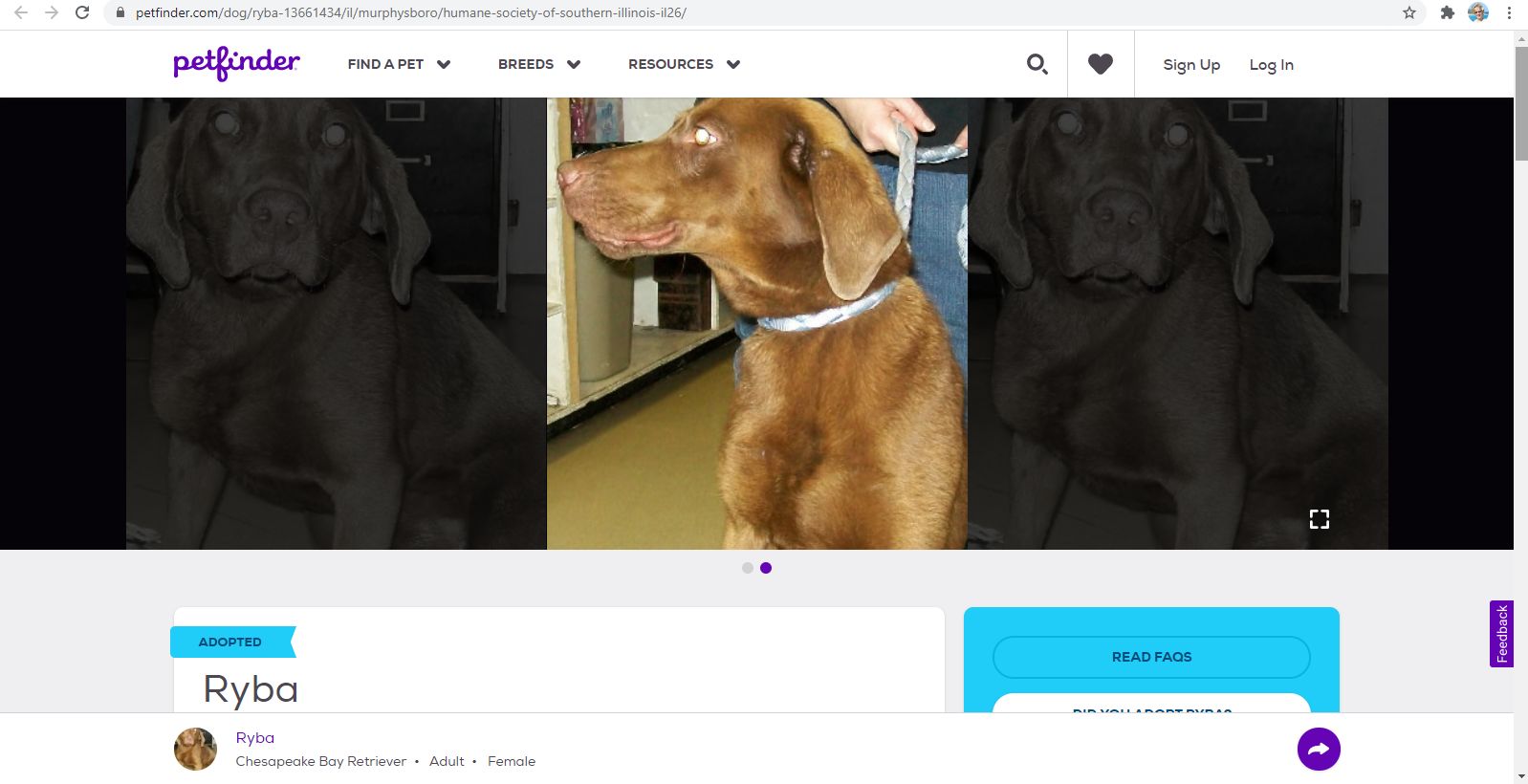This detailed caption describes an image depicting a screenshot of the Pathfinder website:

This screenshot features a webpage from Pathfinder, viewed on a computer, identifiable by the horizontal layout. The browser in use is likely Google Chrome, as suggested by the recognizable interface elements at the top of the screen. The website's name, "pathfinder," is presented in a distinctive purple cursive font on the left-hand side. Adjacent to it are three primary navigation options in black font: "Find a Pet," "Breeds," and "Resources." Further to the right are icons for search (magnifying glass), favorites (heart), "Sign Up," and "Log In."

The main content area focuses on a specific pet. Directly below the navigation categories, there are several photos of a brown dog, prominently featured in the center. The central image depicts the dog facing left, wearing a braided leash held by a person standing behind it. The photo was taken with flash, revealing a slight eye glare. Surrounding this central image are additional pictures of the dog, slightly darkened to accentuate the main photo.

Below the images, a white box displays an adoption status indicated by a blue flag with "adopted" written in blue font. Under this, the dog's name, "Ryba," appears in black font. Further details include an icon of a dog with the text stating, "Chesapeake Bay Retriever, adult female." To the right, a blue box offers a link to "Read FAQs," alongside another button with a share icon within a purple circle, set against a white background.